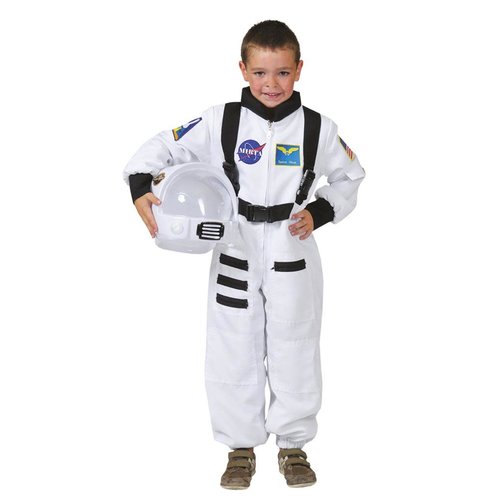This detailed image features a young Caucasian boy, approximately six years old, dressed in a NASA-themed astronaut uniform, possibly for Halloween. The outfit is a white, slightly puffy jumpsuit with intricate black trim on the cuffs, buckles, and belt, as well as black collars around his neck and wrists. Extending to his legs, it has three black stripes on his right thigh and a single black stripe on his left thigh. Prominently displayed on his chest are two emblems: a blue NASA symbol on the right breast and a blue square with gold wings on the left breast. Additionally, there's an American flag patch adorning his left bicep and a triangular blue patch on his right bicep. 

The boy stands confidently, looking directly at the camera with a cute smile on his face. His left hand rests on his hip, while his right arm cradles a white space helmet with a clear visor, situated against his hip. He has short, dark brown hair and brown eyes, adding to his charming appearance. Completing his outfit are brown Velcro shoes. The background of the image is plain white, making the vibrant details of his costume stand out even more.